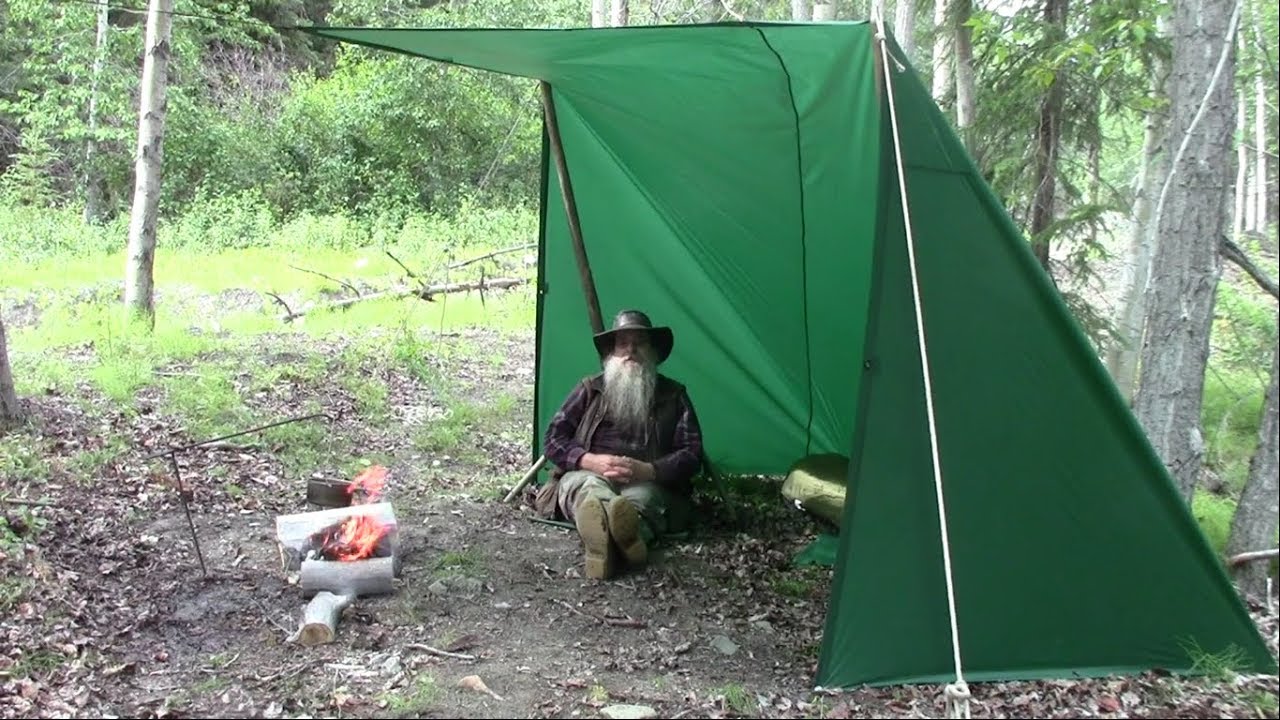A bearded man with a long, white beard is casually seated under a green shelter in the middle of a forest during the daytime. The shelter resembles a half-tent or tarp tent, attached to a tree and partially open, without a bottom floor, providing a temporary refuge. The man, who is wearing a black hat that shades his eyes, along with a brown plaid shirt over another shirt, beige pants, and boots, is positioned against a pole with his legs stretched out in front of him, one foot crossed over the other, and his hands clasped in his lap. He has no discernible expression on his face. To his left, a small fire is burning among some logs, and a pole with a pot hangs near the fire. The immediate area around the shelter is somewhat cleared, but dense forest and foliage fill the background, with sunlight streaming through the trees, casting light on the scene. The ground around the shelter is covered with dirt and leaves, contributing to the rustic, outdoor setting.